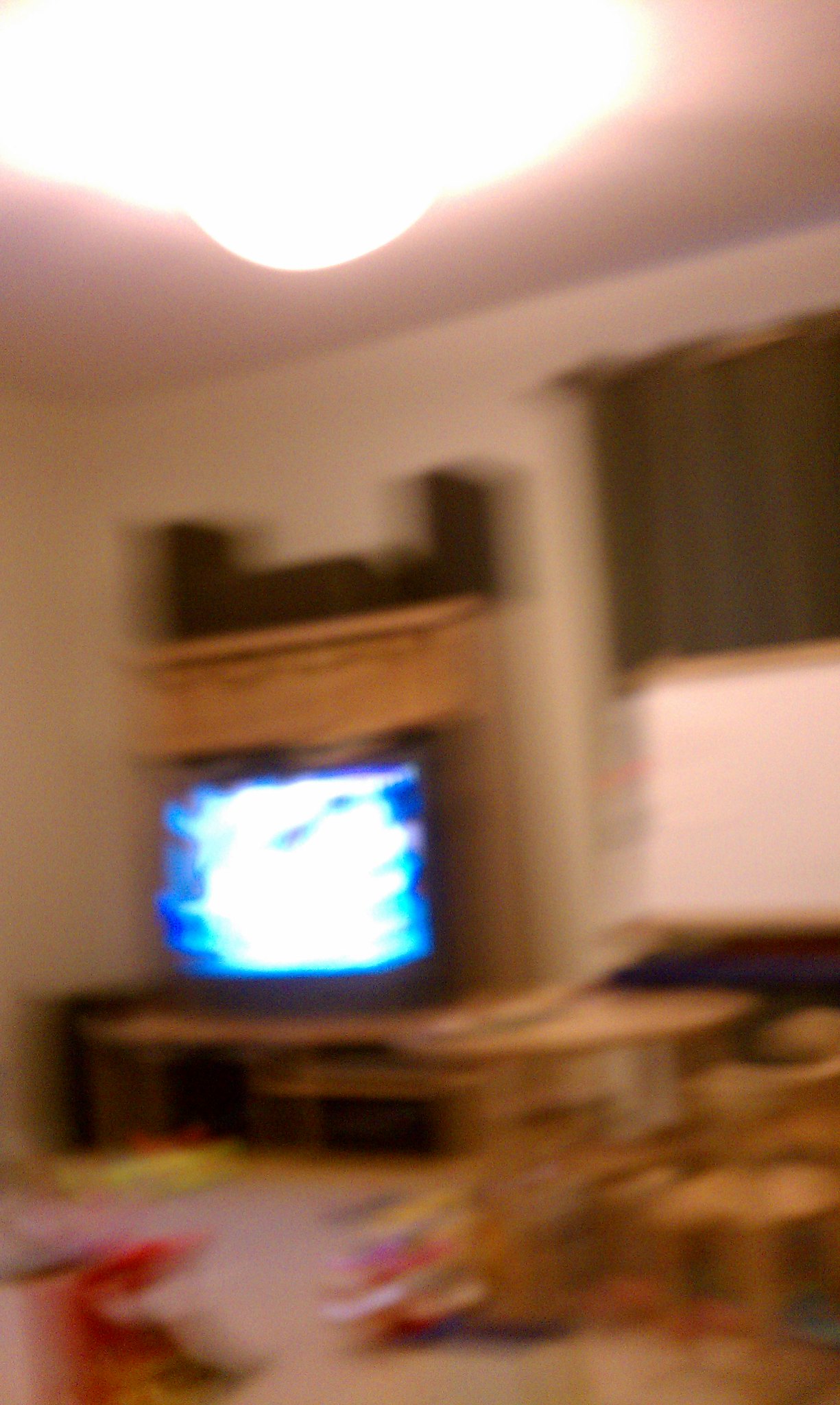This image is an extremely blurred photograph of an interior room, likely a living room, with several discernible features. Dominating the scene is a table or entertainment center made from light-colored wood, housing a turned-on TV whose screen content is indiscernible due to the blurriness. Above the TV, dark shapes that could be a stereo system or another device rest on the top shelf. The wall color appears to be pink, contributing to the overall warm tone of the room. Visible through the blur, there is a window on one wall, covered with a combination of white blinds and a short brown curtain. Other noted elements include toys scattered on the floor, a light fixture on the ceiling emanating bright light, and possible pieces of furniture such as a stool and either a couch or a chair. The carpet is tan, enhancing the cozy ambiance. The room also features a variety of indistinct items, possibly including cardboard boxes and a red object, adding to the cluttered look hinted at in the descriptions.